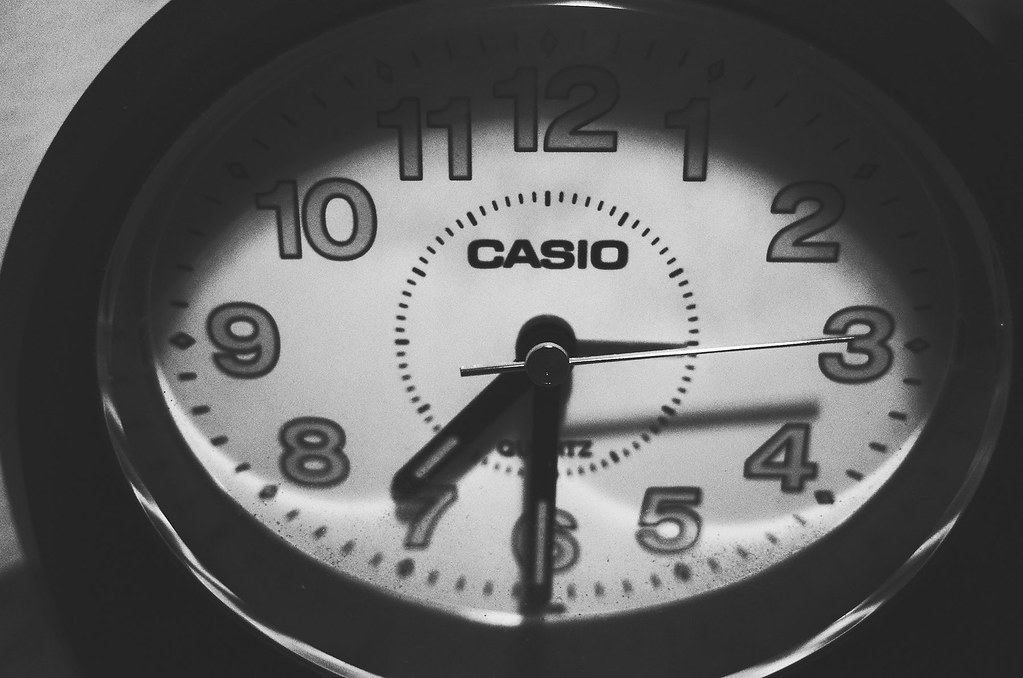A meticulously composed black and white photograph showcases a Casio clock, accentuated by its stark contrast and the subtle shadows of a dimly lit room. Dominating the frame, the clock's outer rim is a deep black, leading the eye inward to a smaller black circle that encloses a pristine white clock face. The numerals, ranging from 1 to 12, are rendered in a soft gray with prominent black outlines, adding depth and legibility.

Encircling the outer edge of the clock face are small hatch marks, serving as minute indicators, with an additional set of finer lines marking the hour increments closer to the center. The time captured in the image is precisely 7:30, marked by sleek, straight black hands with rounded ends, tinged with a hint of gray. The second hand, slender and poised, bisects the clock horizontally, pointing directly at the three.

At the heart of the clock, the brand "Casio" is distinctly printed in black small caps, a testament to its precision craftsmanship. Below the clock hands, within the innermost circle, the label "quartz" can be discerned, though the letters are partially obscured by the hands’ position. This evocative image not only emphasizes the functional beauty of the Casio clock but also captures a moment suspended in time.